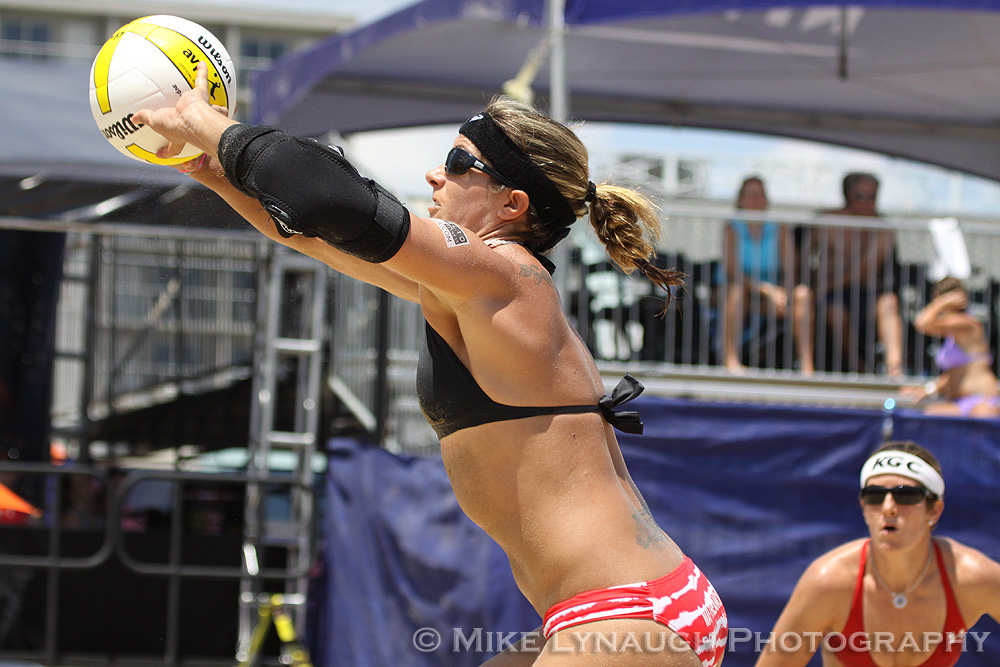In this vibrant outdoor photograph captured by Michael Laino, two women are in the midst of an intense sand volleyball match under the bright sunlight. Central to the image is a white woman with a black headband and dark sunglasses, her brown hair tied back in a ponytail. She is caught in mid-action, her hands extending above her head as she skillfully sets a yellow and white volleyball emblazoned with the word "Wilson." She wears a black long-sleeved top, a black bikini top, and red and white tie-dye bikini bottoms. Small tattoos adorn her back and shoulder, adding to her distinctive look. Her teammate, positioned nearby, sports a red bikini top, dark sunglasses, a necklace, and a white headband labeled "KGC." Behind the players, the background reveals blue tarps and a balcony area filled with spectators keenly watching the game. The photographer's credit, "Michael Laino photography," appears subtly in the bottom right corner of the image, giving credit to this dynamic sporting moment.